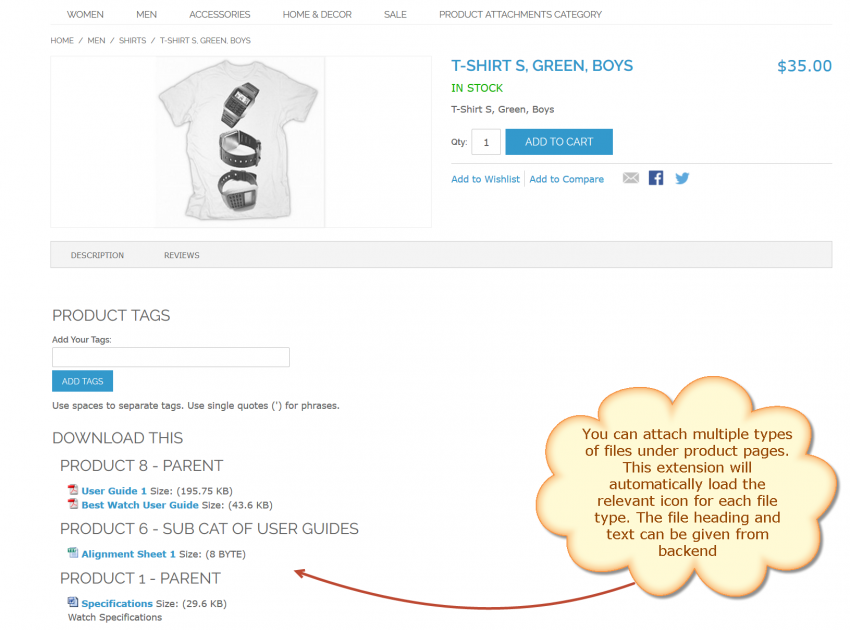Screenshot of a shopping website showcasing a boys' small green t-shirt priced at $35. The item is marked as "In Stock" in green text. Below, the product description reads "T-shirt, Size: Small, Color: Green, Category: Boys" in black text. Customers can select the desired quantity and click the blue "Add to Cart" button. On the left side of the screen, there is an image of the green t-shirt. At the top of the page, the menu bar provides options to browse various categories: Women, Men, Accessories, Home Decor, Sale, and Product Attachments.